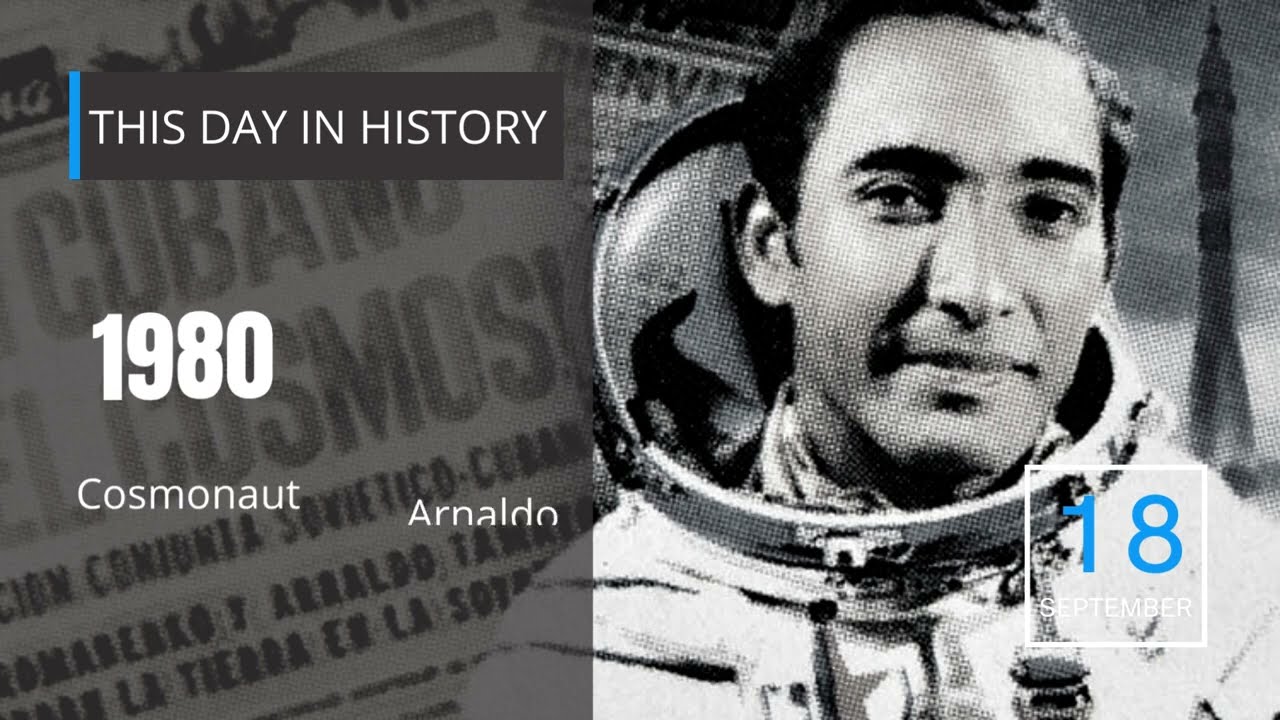This detailed graphic features a black-and-white image of a Cuban cosmonaut named Arnaldo, who is in his late 20s to early 30s. Arnaldo, sporting slightly balding black hair parted to the side and thick, dark eyebrows, has a light smile or slight grin on his face, posing without his helmet in a white spacesuit that includes a distinctive round metal collar. The background on the right side displays a rocket ship, while the left background has a collage of newspaper clippings with a translucent overlay. Visible text includes "This day in history," followed by "1980" and "cosmonaut Arnaldo." The text further mentions "Cubano Cosmo," indicating his Cuban heritage. The bottom right corner features a white square with the date "18 September" in large blue text, marking the historical significance of this date in space exploration history.